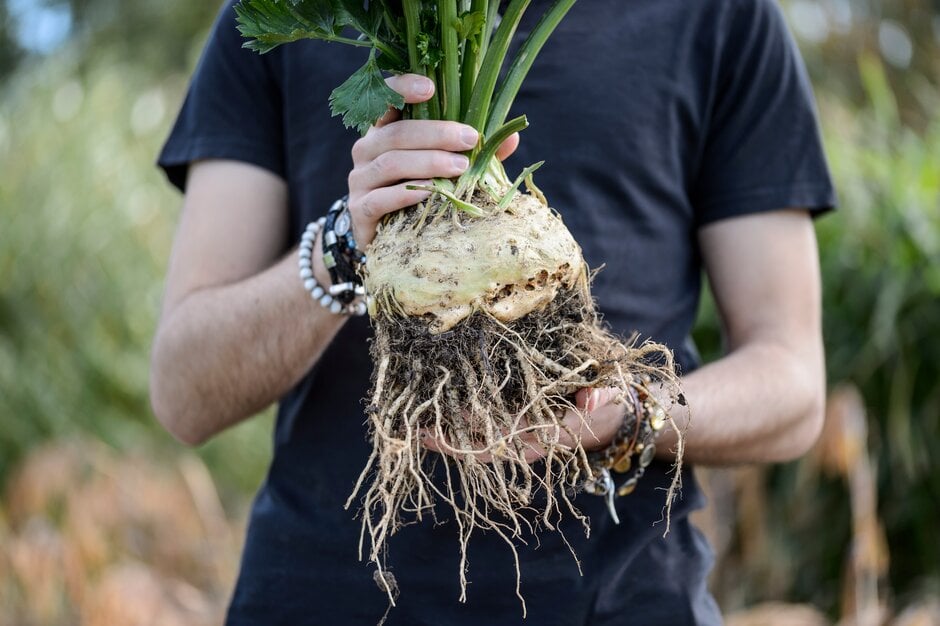In the image, we see the torso and arms of a Caucasian man wearing a dark blue t-shirt and standing against a blurred green background. The main focus of the photograph is on the plant he's holding, which has been uprooted, including its light tan roots. The man's right hand grasps the roots, while his left hand holds the top part of the plant. The plant features white roots hanging down, transitioning into dark green stems. Although the plant appears to be almost like a root vegetable, the exact type is unclear. The man is adorned with several bracelets on his left arm, including two leather bands and a beaded bracelet. The background, though green and suggestive of an outdoor setting, remains unfocused, ensuring that the viewer's attention stays on the uprooted plant and the detailed roots.